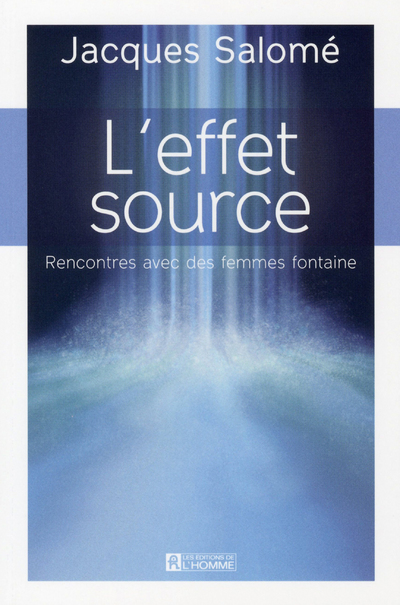The image depicts the cover of a French book titled "L'Effet Source" by Jacques Salomé. The author's name, "Jacques Salomé," is prominently displayed at the top, with an accent above the 'E' in Salomé. The book's title, "L'Effet Source," is written in white text against a blue background that appears to resemble a cascading waterfall. 

Beneath the title, the subtitle "Rencontres avec des Femmes Fontaines" is also in white, suggesting the book discusses encounters with 'fountain women.' The lower portion of the cover features the publication information, "Les Editions de l'Homme," in white text, accompanied by a white logo. The background presents an artistic design that could be interpreted as a tranquil, nature-inspired scene, enhancing the sense of depth and serenity.